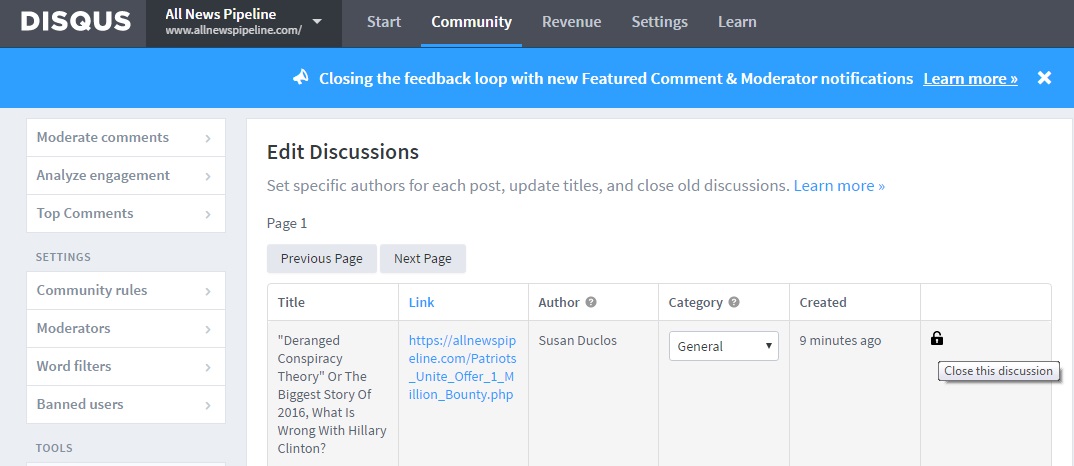This landscape-oriented photo captures the screen of a forum, predominantly featuring the Disqus platform interface. The image is notably wider than it is tall, approximately twice as long as its height. 

At the top, a gray border is delineated by a black line and includes white text. On the far left, "DISQUS" is labeled, followed by a black rectangular box containing the white text "All News Pipeline." Beneath this, the URL "www.allnewspipeline.com" is displayed alongside a drop-down arrow. The submenu options listed are "Star to Community," "Revenue," "Settings," and "Learn," with "Community" highlighted in white and underlined in blue against the gray background.

Below this section, a blue-bordered header stretches from the left-center to the right, featuring white text that reads, "Closing Feedback Loop with New Featured Comment and Moderator Notifications. Learn More," followed by an "X" for closing the notification.

Underneath this header lies a gray column populated with several white boxes. The first white box presents three options: "Moderate Comments," "Analyze Engagement," and "Top Comments." Further below, it lists "Settings," which includes four categories: "Community Rules," "Moderators," "Word Filters," and "Banned Users."

Occupying the remaining space to the right, an "Edit Discussion" box is displayed, filled with various columns in black font. The headings of these columns include "Page 1," "Title," "Link," "Author," "Category," and "Create."

This detailed layout offers a comprehensive view of the user interface elements and functionalities of the forum screen.